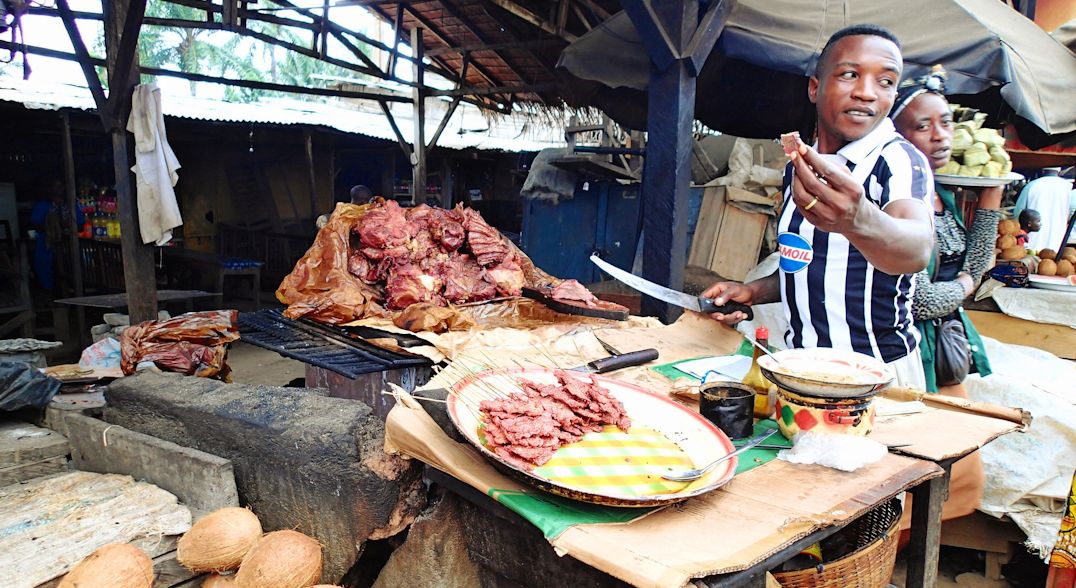In this vibrant color photograph, we see an outdoor market scene, possibly in a tropical or African setting. Central to the image is a man, presumably African or African-American, dressed in a black and white striped shirt resembling a soccer jersey. He stands at a table laden with a large plate of various meats, some of which are on skewers. In his left hand, he holds a piece of meat, possibly offering it to the camera, while brandishing a large knife in his right hand. The man, who is wearing a wedding ring, appears to have just cut the meat from a sizable pile on a stone hearth, suggesting an active cooking area.

Behind the man, a woman wearing an aqua-colored smock and black apron balances a tray loaded with green food items—potentially vegetables or fruit—on her shoulder. Her attire includes a striped black and white shirt, and she glances towards the camera. The setting also features several tables with additional dishes and condiments, possibly soy or Worcestershire sauce. In the dimly lit background, there are lights and what appears to be a jukebox, surrounded by dining tables, indicating this market features both food preparation and dining areas. The scene is bustling, with various meats, bowls, utensils, and even coconuts visible, creating a vivid depiction of a lively and diverse market environment.